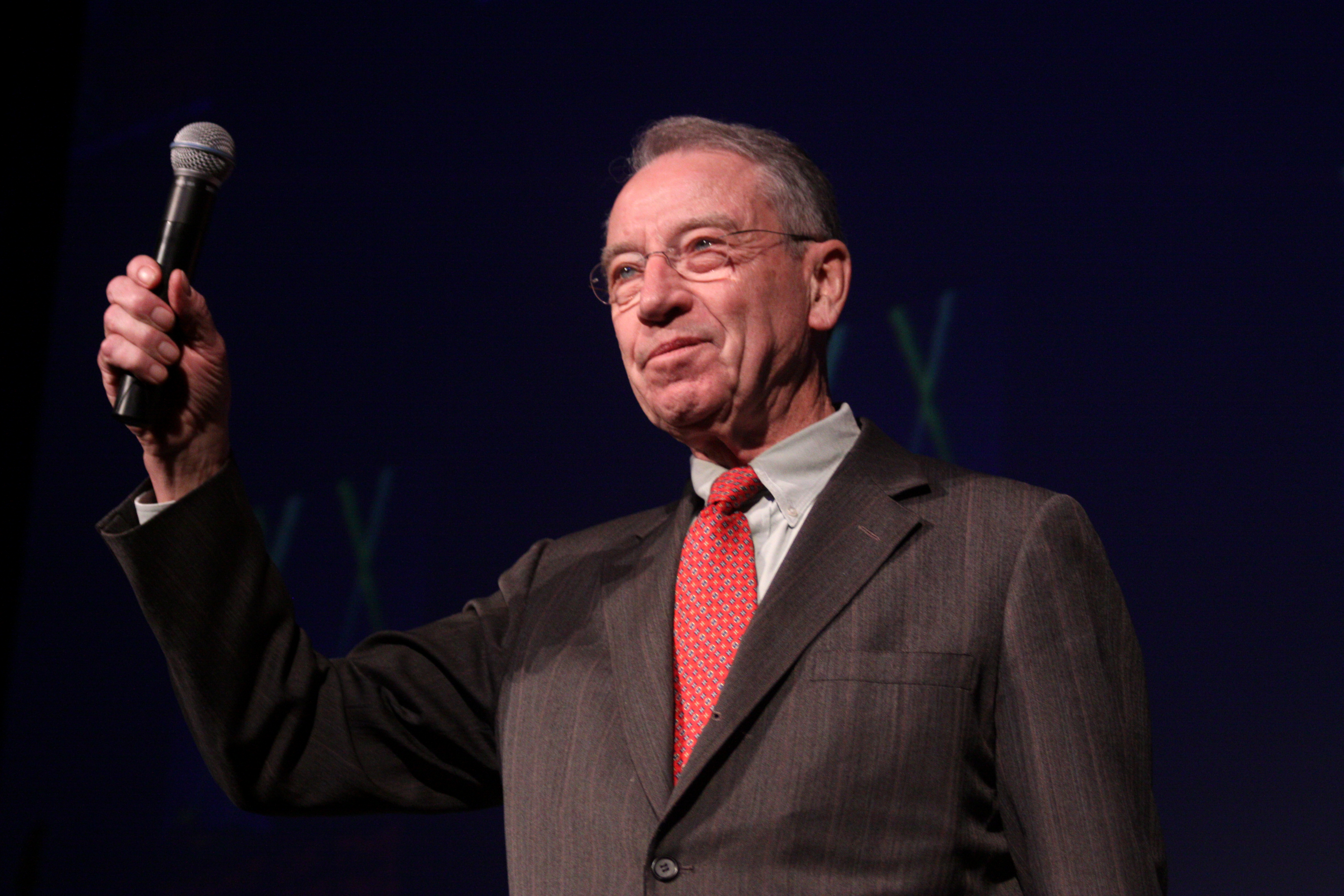The photograph captures a close-up of an elderly Caucasian man, likely in his 70s, who appears to be speaking at an event. His short gray hair sits atop his head, and he wears thin, wire-rimmed glasses. His expression is serious, with a slightly pursed mouth and a wrinkled chin. He is dressed in a dark brown or charcoal gray suit paired with a red tie that features a diagonal diamond pattern and small whitish dots, along with a white collared dress shirt.

The man is holding a small microphone with a black handle and a silver, ball-shaped top in his right hand, raised to eye level and forward, suggesting he is addressing an audience. The background is dark blue and almost completely black, giving an impression of a dimly lit stage. Partially behind him, the faint green glow of letters "YX" or "XXX" can be discerned, possibly from stage signage or a safety outfit. Overall, the image conveys the gravitas of an experienced speaker engaging with his audience.